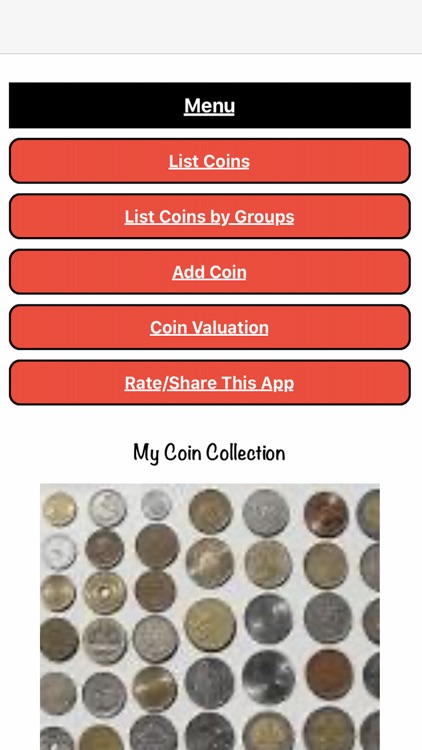The image appears to be a screenshot of a mobile app or website dedicated to coin collecting. At the top, there is a black vertical rectangle featuring the word "Menu" in white, underlined text. Below this, five red banners with white, underlined text display clickable options: "List Coins," "List Coins by Group," "Add Coin," "Coin Valuation," and "Rate/Share This App." Directly beneath these options, the text "My Coin Collection" appears in black. Below this title is a colorful image showcasing six or seven rows of various coins, with different sizes, shapes, and colors. The collection includes bronze, silver, and light brown coins, with one coin notably having a hole in its center. These coins appear to be from different countries and eras, none of them distinctly recognizable as American currency.